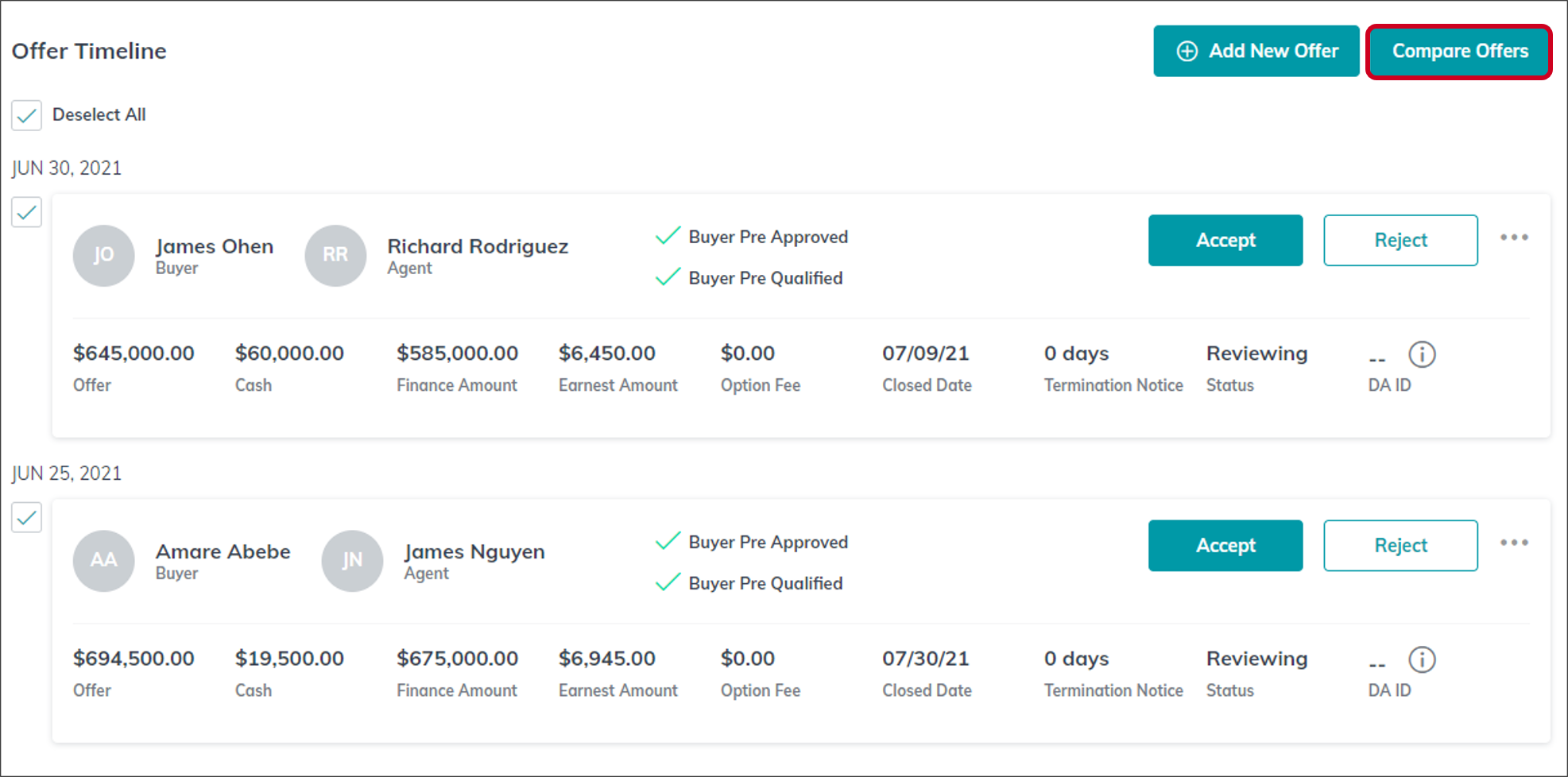This image captures a screenshot from a computer displaying an interface for managing real estate offers. At the top of the screen, there is a title in black text that reads "Offer Timeline". On the left side, there is a teal-colored button labeled "Add New Offer" and another teal button titled "Compare Offers". Notably, the "Compare Offers" button is circled with a red outline, likely to highlight its importance, possibly for instructional purposes in a class or presentation.

The main section of the interface is a detailed offer timeline where all offers are currently selected by default. This section includes columns listing crucial information about each offer, such as the buyer's name, the agent's name, their pre-approval and pre-qualification status, and the ability to accept or reject offers.

In this example, there are two specific entries: one for a buyer named James Ohan and another for a buyer named Amare Abedek Abibi. Both buyers have submitted high offers, and the interface shows options to accept or reject these offers. The red outline around the "Compare Offers" button suggests the importance of this feature in assessing the different proposals.